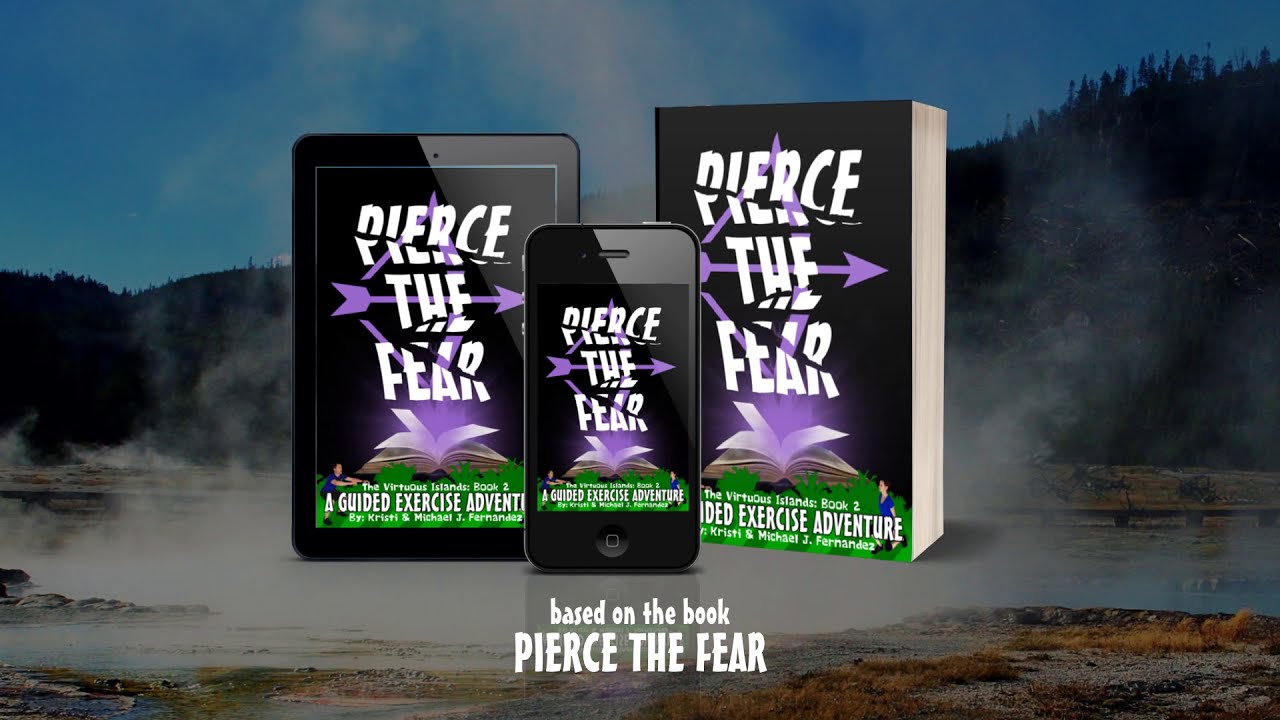The advertisement showcases a serene forest backdrop with hot springs and a large hill on the right side covered in trees. At the center of the image are a book, a smartphone, and a tablet, arranged from left to right. The phone is positioned in front of the other two. All three devices display the title "Pierce the Fear," with a lavender-colored bow and arrow slicing through the text diagonally. Below this, the text reads "A Guided Exercise Adventure," followed by "The Virtuous Island: Book Two" by Christy and Michael J. Fernandez. At the very bottom, in white text, it states, "Based on the book, Pierce the Fear." The background adds to the mystical atmosphere with smoke emanating from the ground and a faint purple hue permeating the scene, suggesting an adventurous and transformative journey inspired by the book.